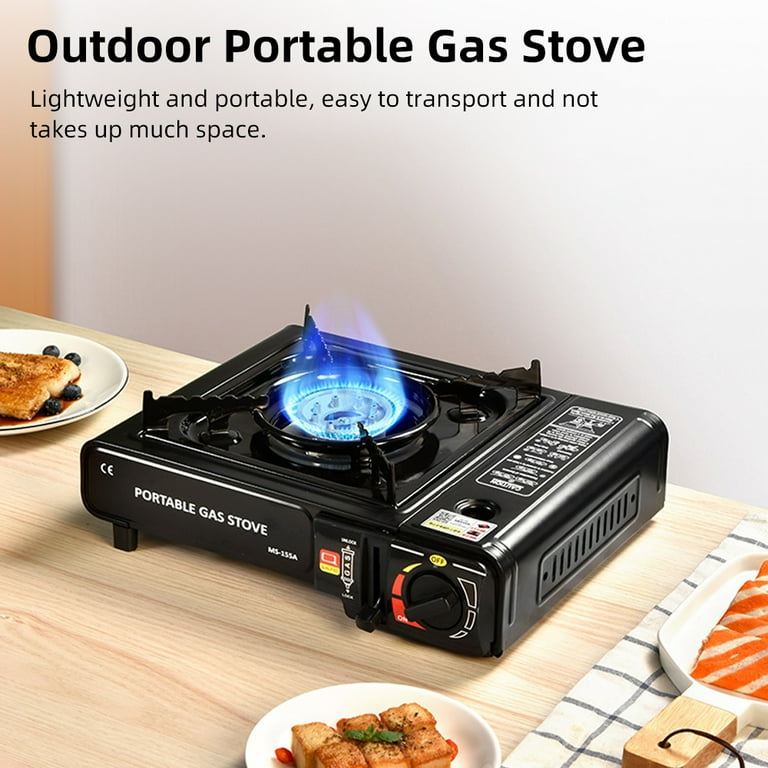Introducing the ultimate outdoor portable gas stove designed to redefine your outdoor cooking experience! This sleek, black stove features a single powerful burner with an impressive blue flame, perfect for any cooking adventure. The compact and rectangular design ensures it sits low on any countertop or table, providing stability and ease of use.

Highlighted by a user-friendly front knob, which adjusts the flame size with precision, this portable stove promises efficient and adjustable heat control. Adorned with a prominently displayed "Portable Gas Stove" label on the front, its elegant black finish seamlessly blends functionality with style.

The advertisement showcases the stove set atop a rustic wooden table, with two white plates of delicious food positioned strategically—one towards the left and one at the bottom center. These plates feature mouth-watering items like tofu and fish, illustrating the stove's versatility in cooking various cuisines.

Above the stove, bold black lettering encapsulates its key features: "Outdoor Portable Gas Stove" followed by "Lightweight and portable, easy to transport, and does not take up much space." This portable gas stove is your perfect companion for outdoor cooking, offering convenience without compromising on performance.